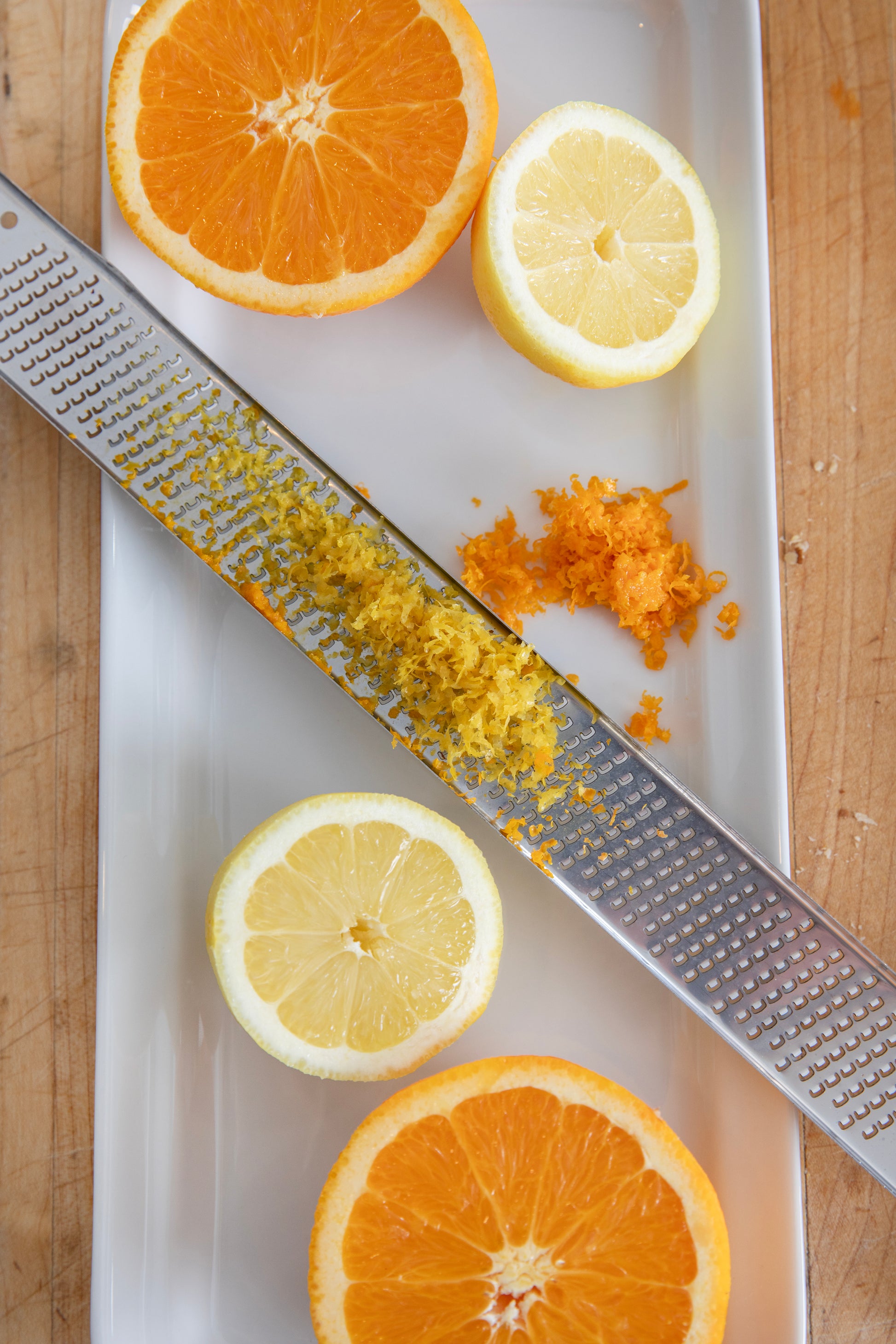The image is a color photograph in portrait orientation, showcasing a white, rectangular platter placed on a beige wooden surface. Upon the platter, a thin, silver microplane grater extends diagonally from the top left corner to the bottom right corner. The grating surface of the microplane displays residues of lemon zest, indicating recent use. Positioned on the platter are various citrus fruits: in the top left corner, a partially cropped, dark orange half of an orange, and slightly lower to its right, a light yellow half of a lemon facing top-right. Below the grater on the left side is another half of the lemon, and at the bottom right, another half of the orange is partially cropped at the bottom. Surrounding the microplane are grated piles of orange and lemon rind, suggesting the fruits were recently zested. The detailed arrangement of the citrus fruits and grater, along with the precise depiction of the colors and texture, exemplifies photographic representational realism.